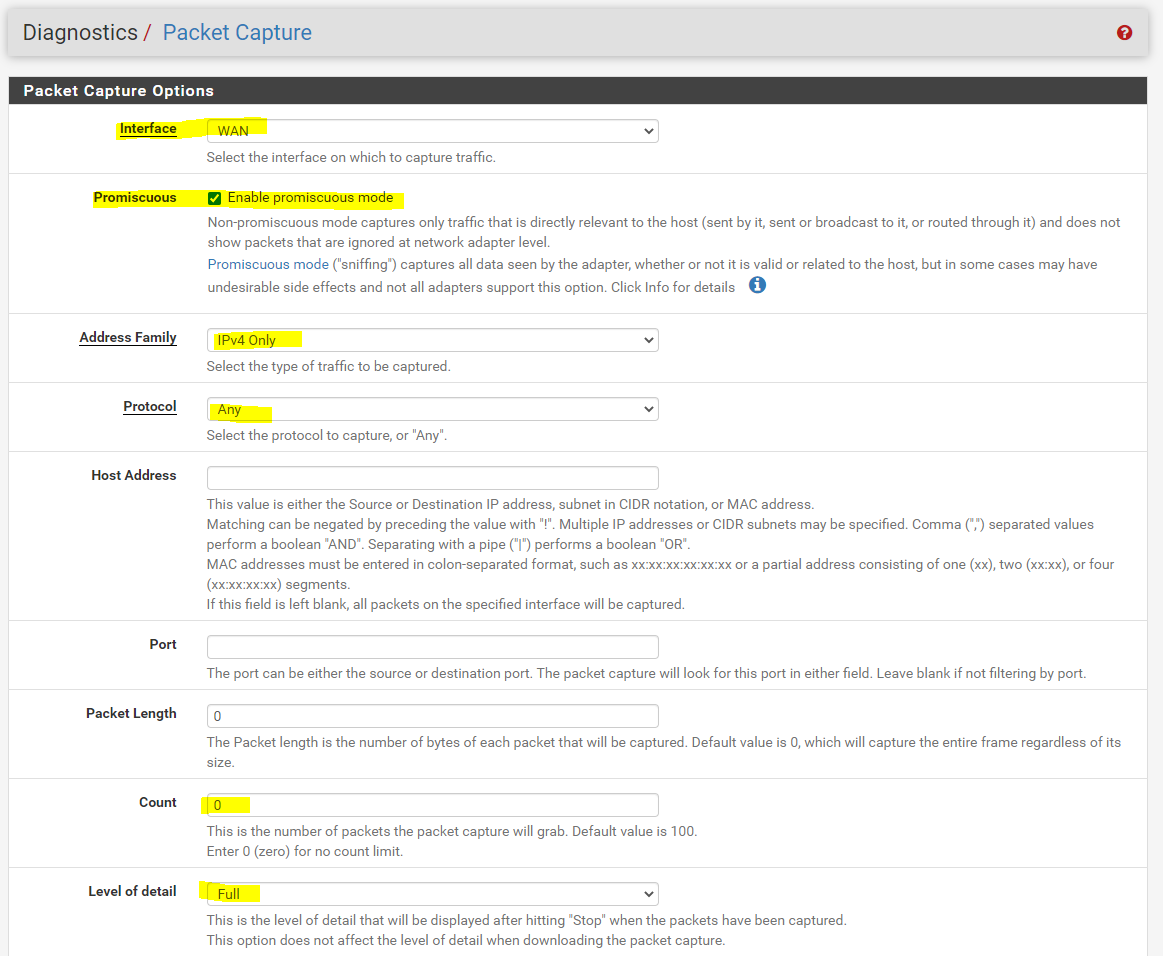The image depicts a white web interface with predominantly black text. At the top, there is a gray bar featuring the title "Diagnostics / Packet Capture" in a mix of black and blue fonts. Adjacent to the title is a red circle with a white question mark inside it.

Beneath the gray bar, a black tab labeled "Packet Capture Options" in white text is visible. The interface continues with several highlighted sections outlined in yellow:

1. **Interface WAN**: Displays a dropdown menu where users can select the interface on which to capture traffic. The description states, "Select the interface on which to capture traffic."

2. **Promiscuous Mode**: This section includes a green and white checkbox labeled "Enable Promiscuous Mode." The accompanying description explains that in non-promiscuous mode, only packets directly relevant to the host are captured. Promiscuous mode captures all data seen by the network adapter, though this mode may have undesirable side effects and is not supported by all adapters. Users are prompted to click "Info" for further details.

3. **Address Family**: This dropdown menu defaults to "IPv4 only" and allows users to select the type of traffic to capture.

4. **Protocol**: Another dropdown menu labeled "Any" lets users select specific protocols for traffic capture.

5. **Host Address**: Accompanied by a blank white input box, this field accepts the source or destination IP address, subnet in CIDR notation, or MAC address. The description notes that negation can be done by preceding the value with a character. Boolean operations can be performed by separating multiple IP addresses or subnets with a pipe symbol. MAC addresses must be entered in a colon-separated format. Leaving this field blank captures all packets on the specified interface.

6. **Port**: This field, currently empty, accepts either the source or destination port. Leaving it blank will not filter the capture by port.

7. **Packet Length**: Set to zero by default, this field specifies the number of bytes in each packet to be captured. The default value captures the entire frame regardless of size.

8. **Count**: Highlighted in yellow, this field is set to zero. It represents the number of packets to capture, with a default value of 100. Entering zero indicates no count limit.

9. **Level of Detail**: Also highlighted in yellow, this dropdown menu allows users to select the level of detail to be displayed after stopping the capture. This setting does not affect the level of detail for downloaded captures.

The interface is clearly designed for detailed packet capture configuration, with various options for customizing the scope and depth of captured network traffic.